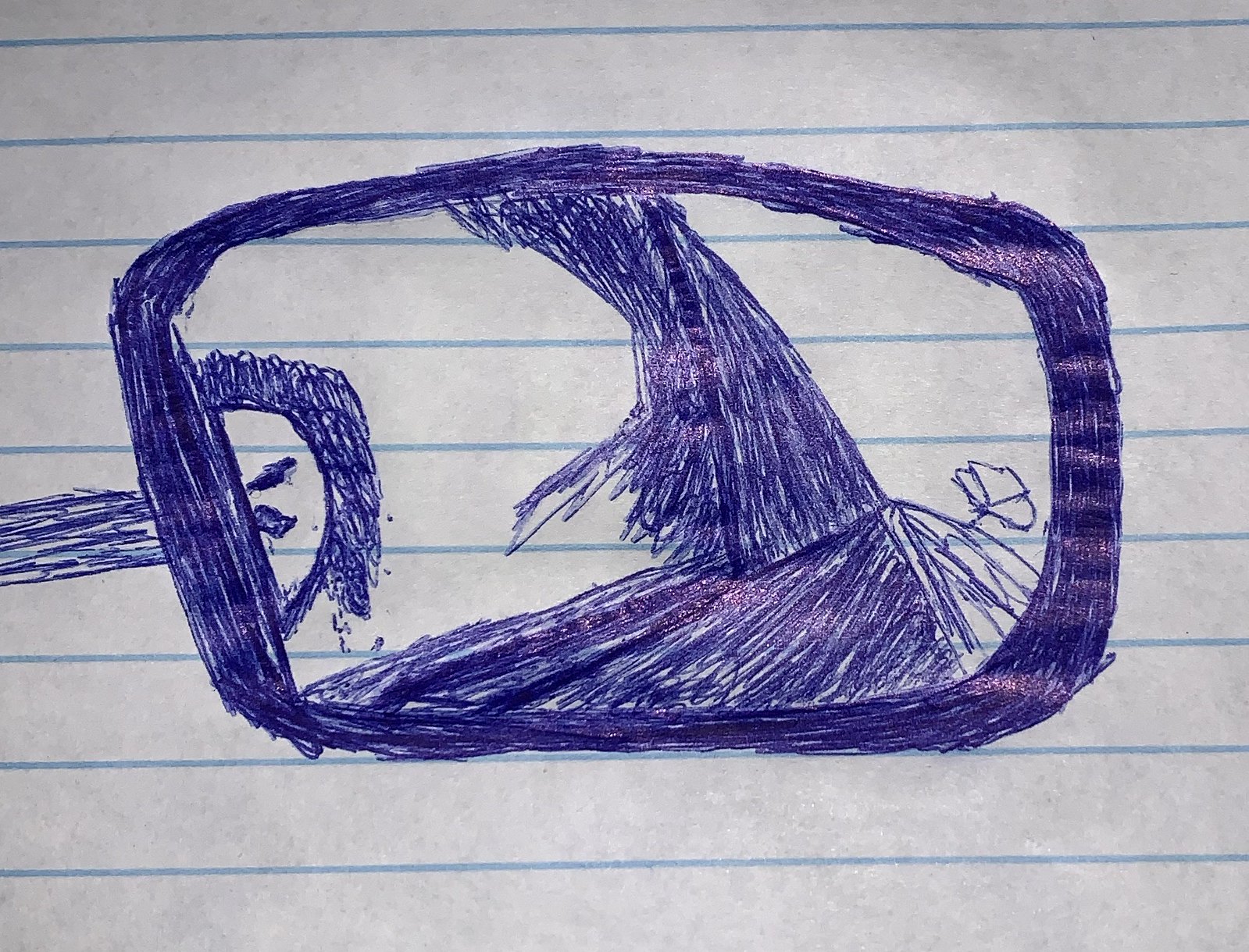The image depicts a detailed ink pen doodle on a sheet of white notebook paper, characterized by evenly spaced blue lines. The central element of the drawing is a thickly bordered, oval-shaped form, presumably created by repeatedly circling with a heavy ink pen. Emerging diagonally downward from the bottom of this oval is a roadway-like path that branches out into a pyramid or triangular shape towards the top of the page. 

On the left side of this central oval is a thin portion leading into the oval and a semicircle with two lines inside it. Additionally, there appears to be a rectangle with heavily inked borders on the side, and a small semicircle atop this border, resembling a head with curly hair and two eyes. The detailed drawing within the oval suggests a scene possibly resembling a right side mirror of a car, showing the reflection of an angry man with thick hair and a mustache in the passenger seat. Despite its incomplete appearance, the doodle intricately merges abstract and identifiable elements.